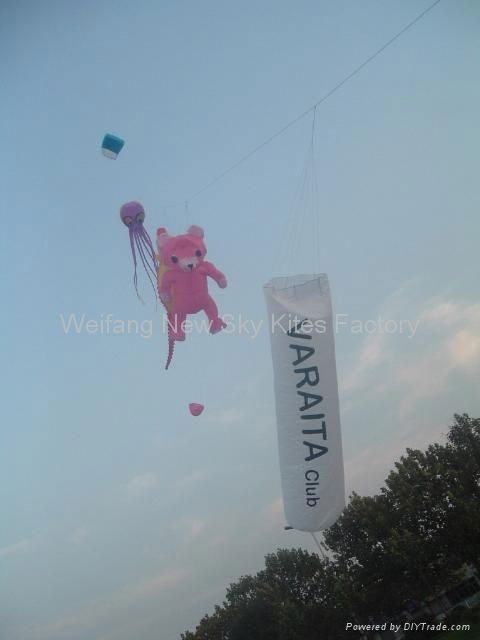In this outdoor image, against a light blue sky adorned with soft, wispy clouds, various kites hang from a thin wire strung high above. Dominating the visual scene is a large rope extending diagonally with an assortment of kites attached. The highest floating kite resembles a traditional parachute. Below it, a vibrant purple octopus kite with slender arms dangles in mid-air, subtly positioned to the upper left. Close to the center, a larger-than-life pink and white teddy bear kite, detailed with a white snout, black eyes, and black nose, sways gently. Adjacent to the bear, a tall rectangular banner kite, featuring the bold, capitalized inscription "VARAITA" followed by the smaller word "club," flutters in the breeze. Anchoring the scene, a dark green tree sits in the bottom right corner. The image is subtly branded with a watermark reading "Weifang New Sky Kites Factory," and in the lower-right corner, there's a mark stating "powered by DIYtrade.com." The colors throughout the image vary from shades of blue, turquoise, and white to bursts of purple, pink, and green, creating a lively, dynamic display against the serene sky.